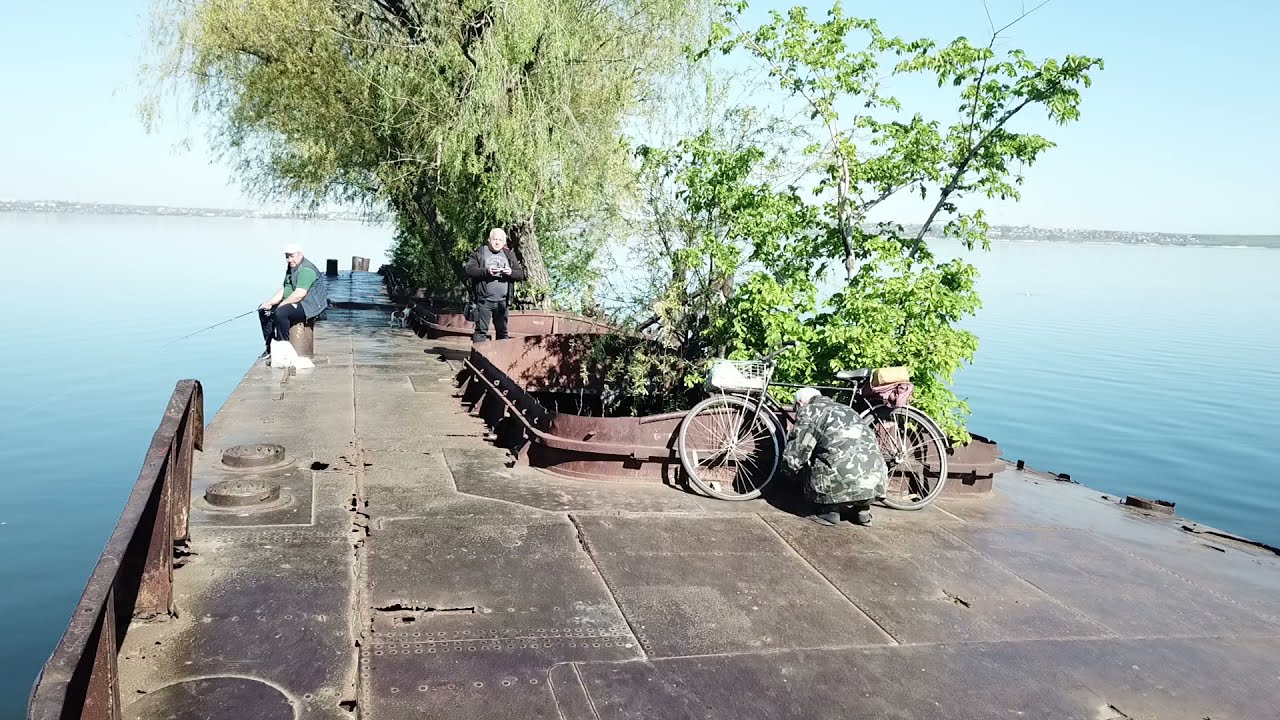This photograph captures a breakwater structure extending into a vast, blue sea. The structure is constructed from large, rectangular sheets of concrete and metal, with a rusty, gray, and brown ground. In the center of the breakwater, there are metal-framed planters housing tall trees, including a lush, green willow. The horizon reveals distant land with faint foliage and buildings.

In the scene, three individuals are positioned at different points of the breakwater. On the left, a man sits on a post, holding a fishing rod over the edge, engaged in fishing. In the middle, a person dressed in a camouflage coat bends down, repairing a bicycle propped against one of the planters. More centrally, another man, clad in black, stands and looks towards the camera, his hands held in front of him. The vibrant greenery of the surrounding plants adds a serene contrast to the industrial materials of the breakwater against the backdrop of the tranquil, blue expanse of the sea.